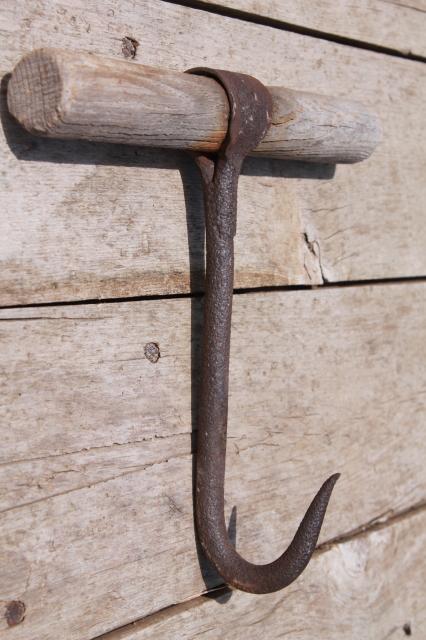In this detailed close-up photograph taken inside a shed or similar wooden structure, the focal point is a large, rusty metal hook with a thick bottom that curves upward into a longer, straight segment. This segment passes through a ring and suspends a rounded wooden handle. The hook likely evokes historical tools used for butchering meat or preparing jerky. It is securely mounted on a section of the wooden wall planks, which are weathered and marked by rusty nails and subtle dot markings. The hook itself appears very sharp and is firmly attached to what seems to be a third vertical slat of the wood wall background, all of which share a typical brown hue, blending seamlessly together.